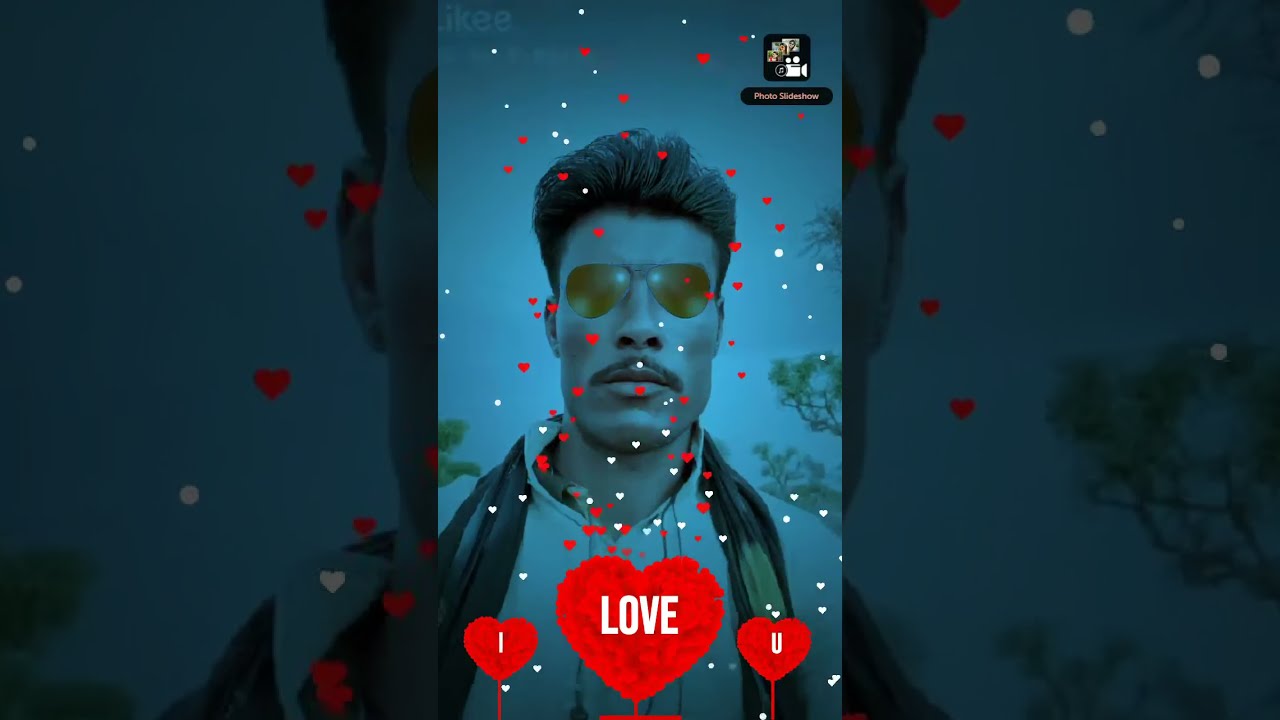In this image, we see a man with dark hair, combed over to the right, and a handlebar mustache, looking slightly downwards with a faint scowl. The entire image has a blue hue, likely due to a filter, and is filled with various red and white heart shapes of differing sizes. The man appears to be the focal point, positioned centrally within the frame, giving the impression that this may be a selfie overlaid with decorative elements.

At the top right corner, there is a black emblem featuring a white camcorder icon along with the text "Photo Slideshow" also in white. Below this, three larger hearts dominate the lower central area of the image. These hearts spell out the phrase "I love you," with the heart containing "love" being the largest and centrally positioned. The other two hearts, "I" and "you," flank it on the left and right, respectively. Scattered throughout the image are numerous smaller red and white hearts, enhancing the romantic theme.

Overall, the composition combines both drawn and photographic elements, including some white-drawn mountains and a blue sky in the background, adding to the layered visual effect. The coordinated colors, with red and white hearts against a blue hue, create a visually striking and emotive image.